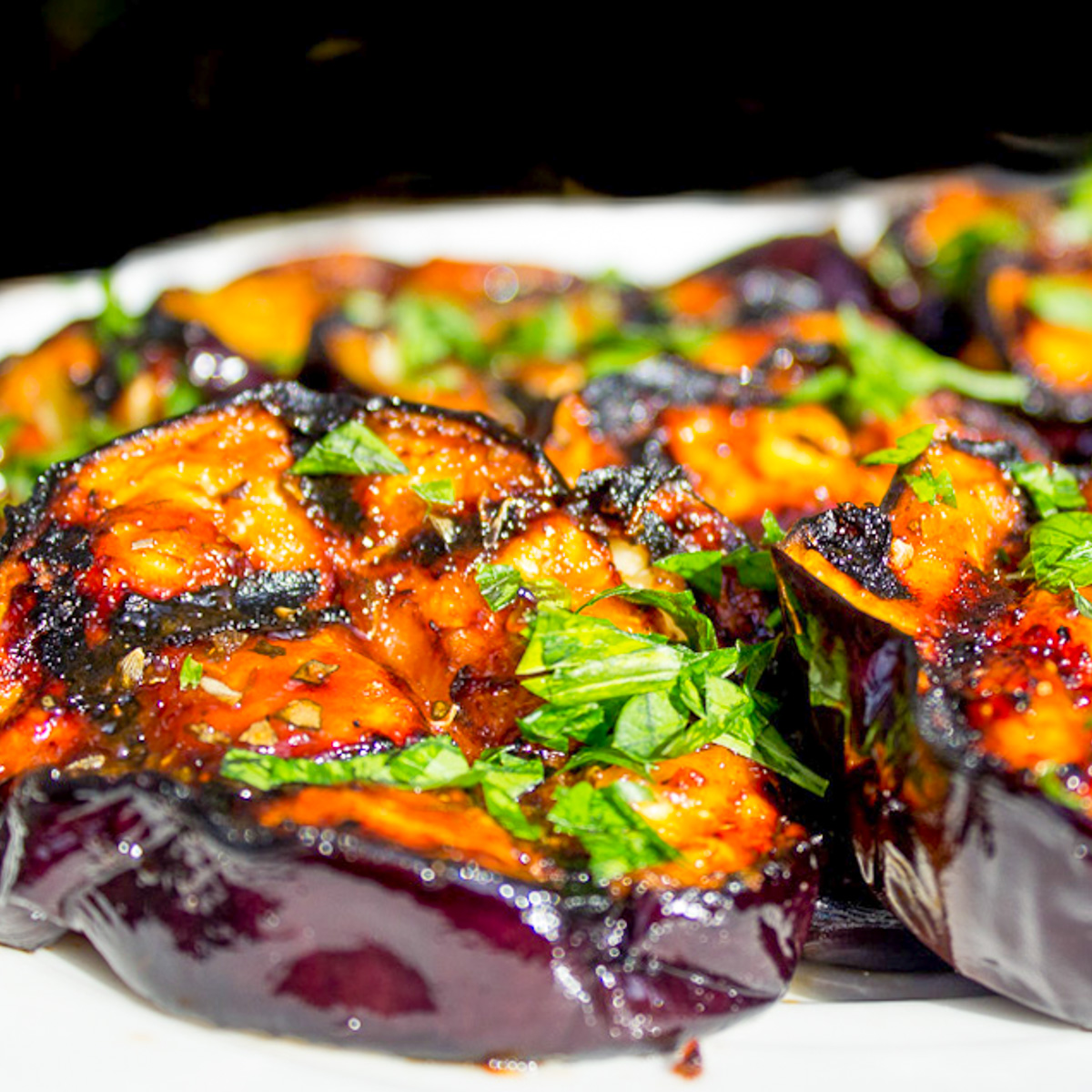This very detailed close-up photograph features a meticulously arranged plate of food. The white plate, visible only in the lower right and upper portions of the image, serves as a subtle backdrop to the main focus: circular slices of grilled eggplant. The eggplant pieces, which dominate the frame, boast distinct grill marks and their flesh exhibits a rich orangish-yellow hue, suggesting a glaze or sauce has been applied. An artistic trim of shiny, burgundy-red sides enhances their polished appearance. Finely chopped lettuce, scattered across the eggplant, adds a touch of vibrant green, contrasting beautifully with the golden gleam of the glaze. The depth of field effect keeps the background slices blurred, emphasizing the foreground details and creating an evocative visual narrative of this gourmet presentation.